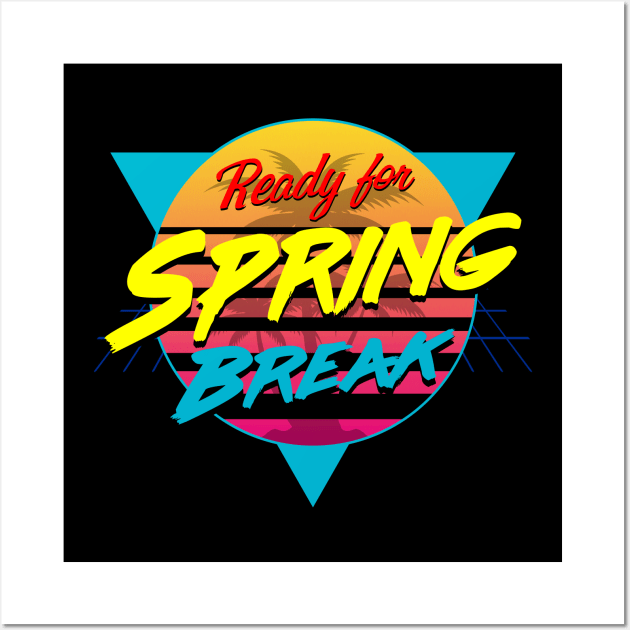The image is a square with a white border surrounding a black background. Dominating the image is an upside-down teal triangle occupying approximately two-thirds of the space. Superimposed on the triangle is a large circle featuring a striking gradient effect that transitions from bright orange at the top to hot pink at the bottom. This circle is adorned with several palm tree silhouettes in light grey, adding a tropical flair. Black lines traverse the middle of the circle, creating a sense of texture and depth. At the top of the circle, in red script font, are the words "READY FOR." The central, most prominent element is the word "SPRING" in bold, bright yellow, extending across the middle of the circle. Below that, in the same teal as the triangle, the word "BREAK" is written in a thick, handwritten-style font. The vibrant colors and dynamic composition evoke a sense of excitement and anticipation for a tropical spring break.